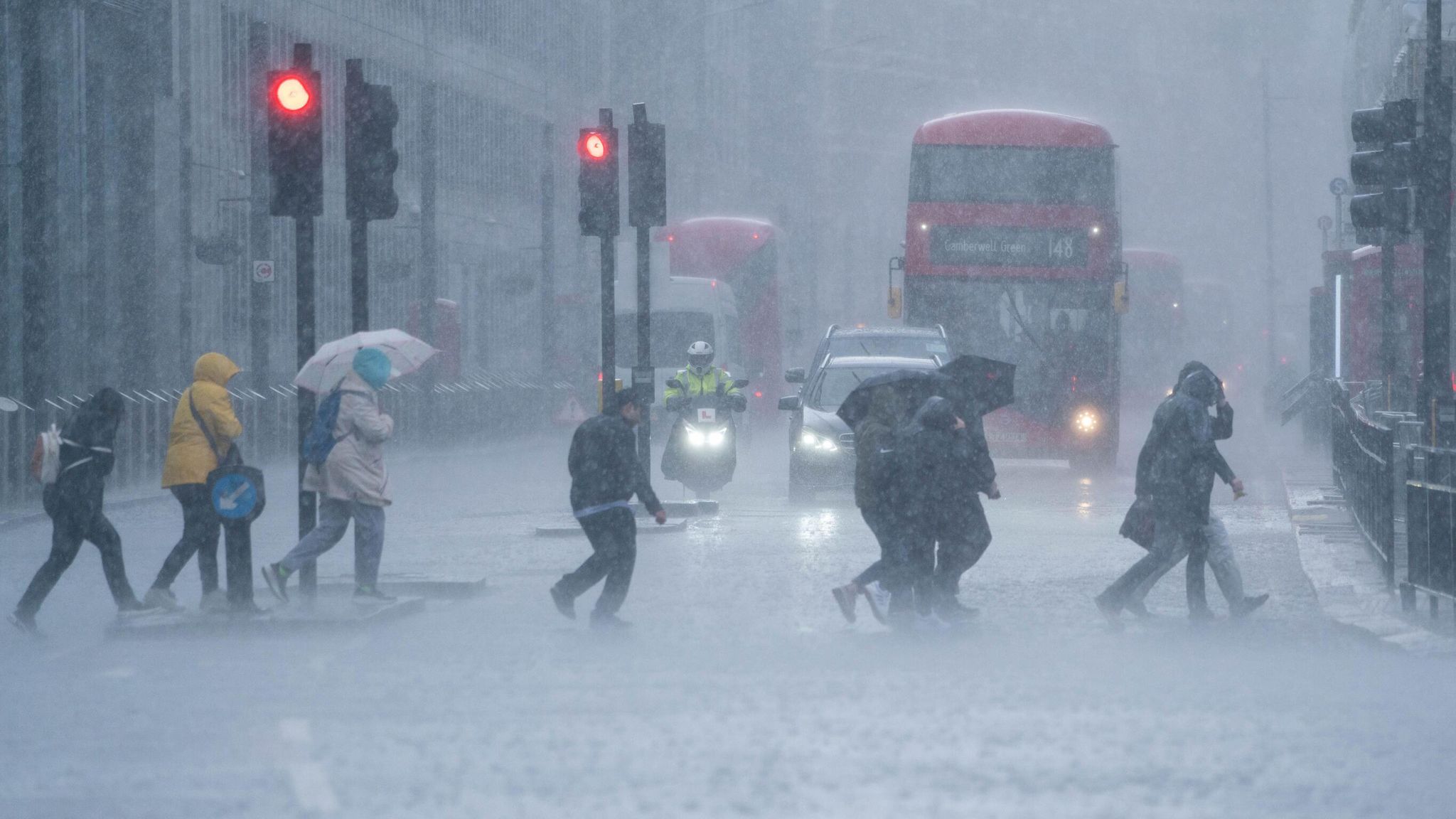The photo captures a rainy day in what appears to be London, England, identified by the iconic big red double-decker bus in the background. Approximately ten people are braving the heavy rain, crossing a city street at a red light, with most of them wearing jackets and a few sheltering under umbrellas. The scene is dominated by the overcast, dimly-lit sky which casts a gray hue over the surrounding buildings and streets. The ground is slick with rainwater, and the cars lined up at the intersection have their headlights on, enhancing the sense of a dreary, rainy day. The backdrop also includes various other vehicles, such as a motorcycle and several cars, all stopped at the red light, their lights glowing through the downpour. The urgency of the pedestrians, some with raised hoods, as they hurry across the wet street, vividly captures the essence of a typical rainy day in a bustling city.